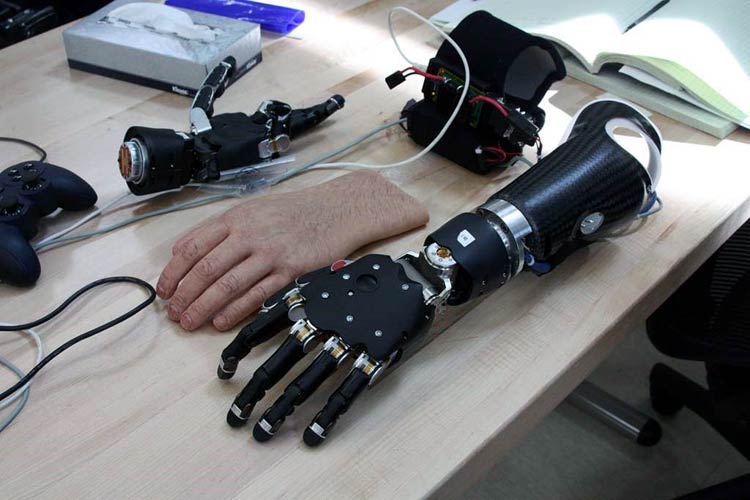The image depicts a well-organized work table in what appears to be an office or lab environment, distinguished by a sleek, modern wooden surface and a silver metal frame. In the foreground on the right-hand side, sits a sophisticated black robotic hand, composed of metal or black carbon with prominent silver joints at the wrist, base of the fingers, and nails. This mechanical hand is closely juxtaposed with a highly detailed, life-like prosthetic model of a human hand, designed to resemble Caucasian skin, likely made from latex. 

Adding to the assortment on the table, there are various essential items: a rectangular box of tissues with white tissues emerging from its center, an open but unreadable notebook, multiple colored cables and wires, and an indispensable console controller. Notable too is a power supply or an unspecified kit that plays a crucial role in the scene. The presence of a chair in the foreground and a box of latex gloves in the upper left corner solidifies the setting as operational rather than merely decorative. This collection of objects and the methodical arrangement hint at an active workspace engaged in advanced prosthetic or robotic development.